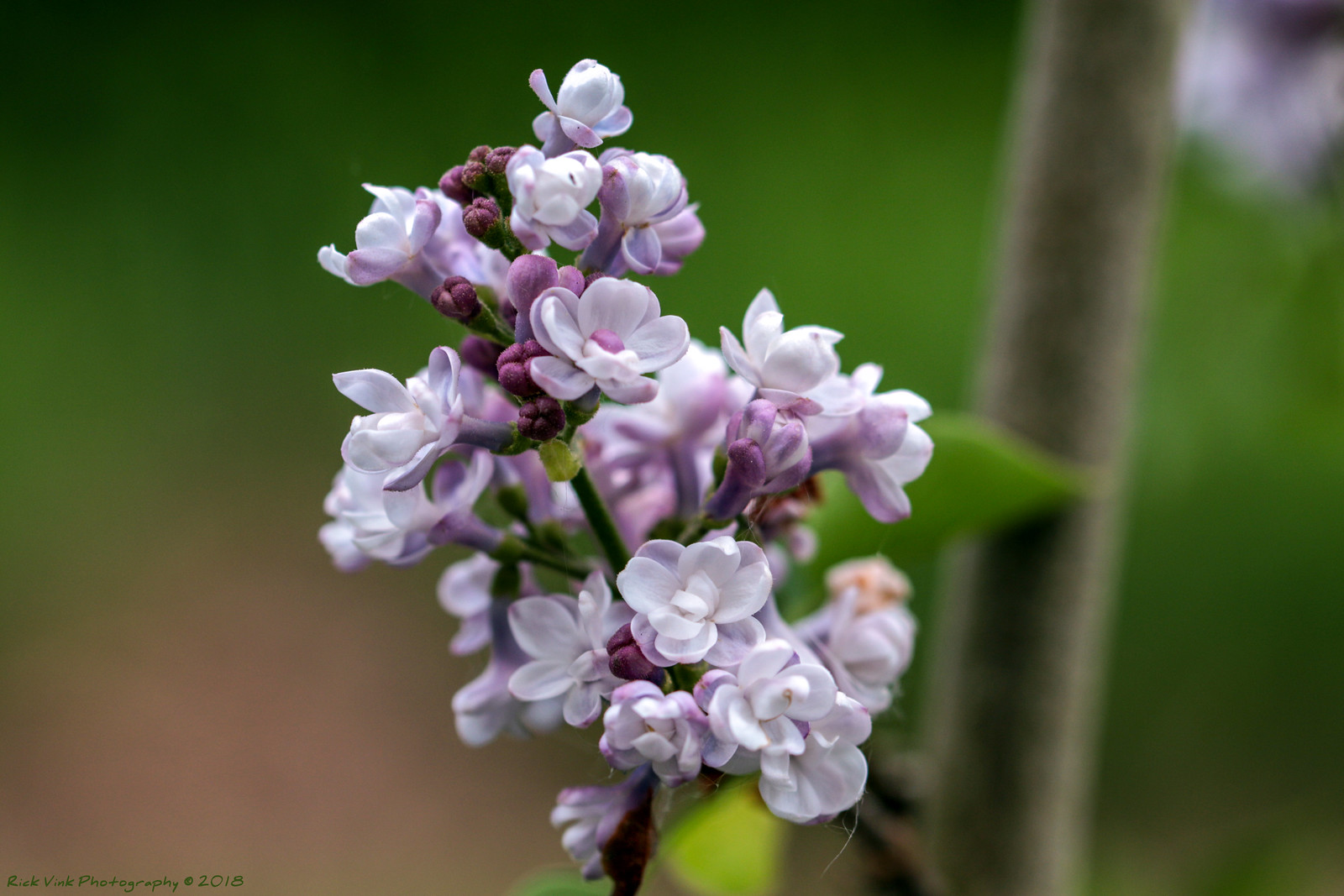The image is a horizontally aligned rectangular close-up of a small flowering plant, captured in sharp detail against a blurred, green background likely consisting of grass or other plants. The central focus is on delicate flowers with lavender petals interspersed on a green stem. Some flowers are fully blossomed, revealing white petals tinged with purple on the edges, while others are still in the bud stage, displaying a darker purple hue. The green stem ascends from the lower part of the image toward the center before fading into the blurred background. In the bottom left-hand corner, there is a small, green font inscription that reads "Rick Vic Photography © 2018." Additionally, a grayish-brown pole is visible along the right side of the frame, extending from the bottom to the top of the image against the out-of-focus greenery and a hint of brown which might be a sidewalk or dirt patch.